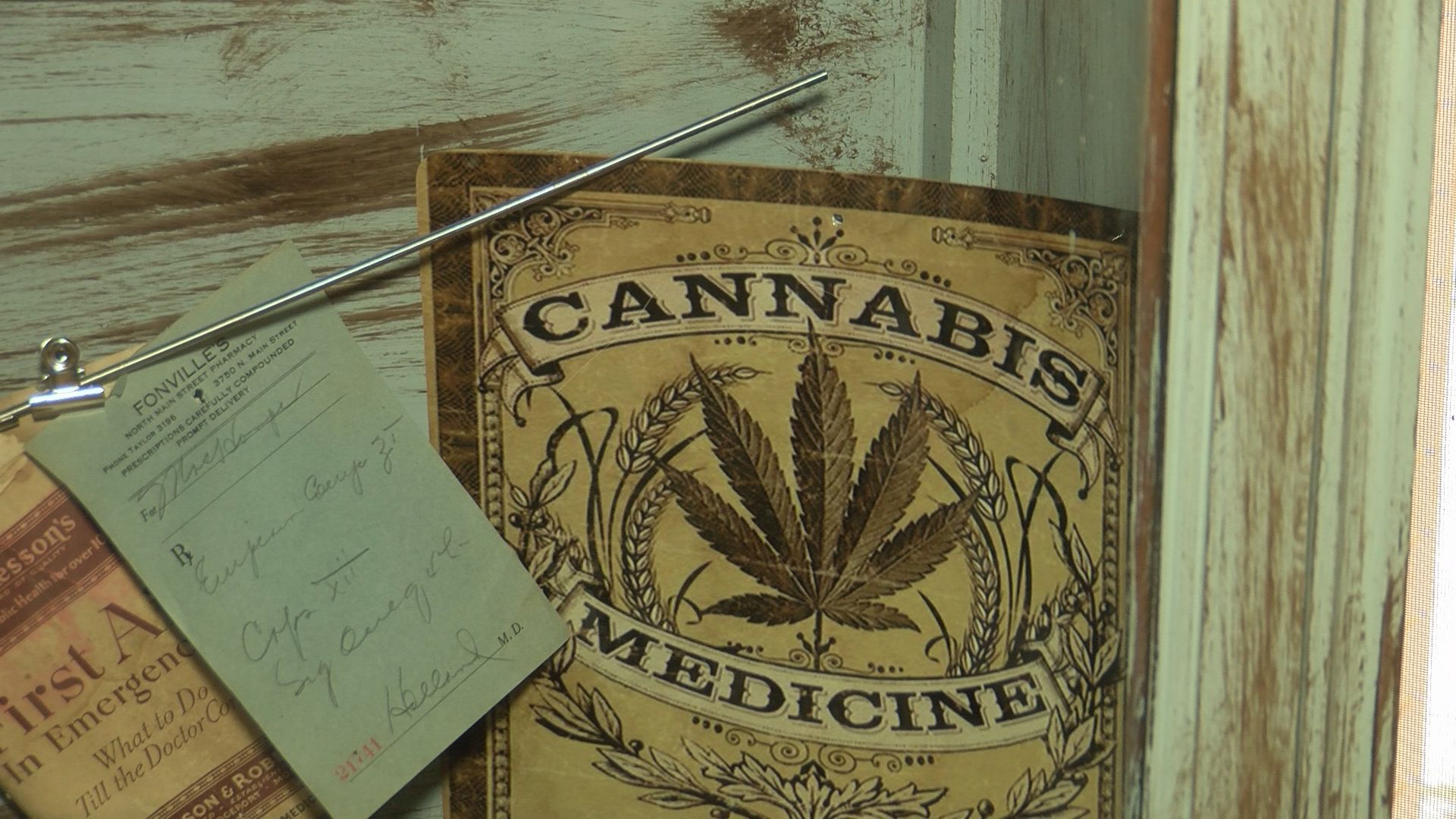The image features a rustic, distressed wooden wall, painted in a fading lime green color that reveals natural wood beneath the paint. Attached to the wall are three papers. The first piece of paper reads "Cannabis Medicine" and prominently displays a stereotypical seven-leaf marijuana plant, accompanied by two pieces of wheat arching around the central leaf. The design is rendered in shades of brown, black, and beige. Adjacent to this is what appears to be a prescription held in place by a slim metal rod with a clip. The prescription is from Fawnville Pharmacy, includes detailed instructions, a signature, and a number at the bottom. Below this, a third paper is partially visible, with text that starts with "First Aid in Emergency." The setting suggests an old medical dispensary, housed in a historically styled building with weathered interior decor.